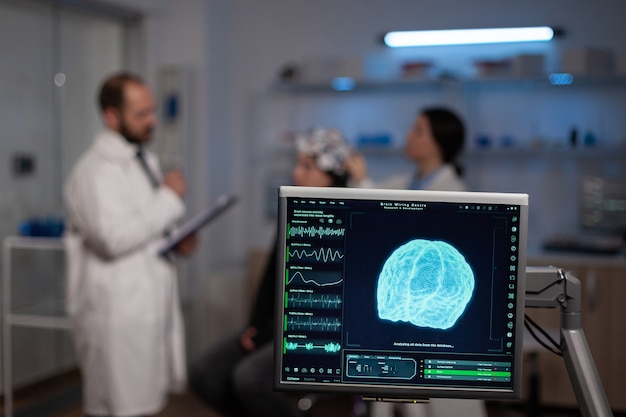In a pristine, white-walled doctor's office, the scene unfolds around a central piece of advanced medical equipment. The foreground features a highly focused video screen displaying a blue-tinged, illustrated scan of a brain, complete with frequency and volume-styled lines reminiscent of an EKG readout on the left side, and boxes of text, albeit illegible, on the right. The background, slightly blurred, reveals a balding white male doctor with a beard and glasses, dressed in a white lab coat. Holding a clipboard in his right hand, he seems poised to jot down notes. Opposite him stands a white female doctor, also in a white coat, partially obscured by the foreground screen. She appears to be manipulating a white contraption placed on the head of a patient seated between them. The patient, whose gender is indistinct, is fitted with a device that might resemble tinfoil, suggesting it’s used for brain imaging or monitoring. Behind the group, metallic shelves are stacked with storage boxes, illuminated by a fluorescent blue light above. The room’s clinical, well-organized environment highlights the professional and focused nature of this medical evaluation.